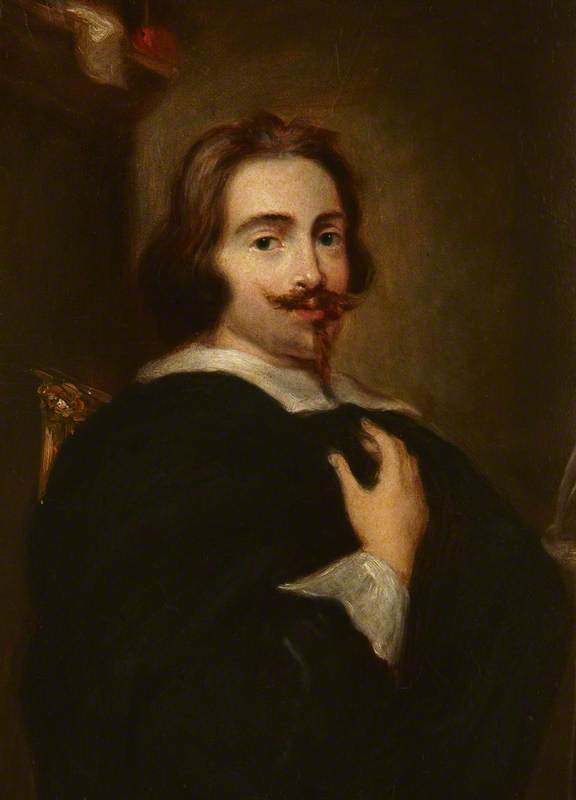The painting, reminiscent of the style of the Grand Masters, depicts a young gentleman seated on an intricately carved wooden chair, partially visible in the frame. The man, aged perhaps in his late 20s to early 40s, has shoulder-length brown hair that blends subtly with the muted background of browns and greenish grays. His face is chubby with thick eyebrows, big brown eyes, and a characteristic handlebar mustache curling upwards, complemented by a thin goatee extending from his lip below the chin.

Draped in a black robe indicative of historical or legal attire, he sports a distinctive square-shaped white collar and prominent white cuffs at his wrists. His right hand rests on his chest in a pensive pose. The background is largely non-descriptive, save for hints of a mantle or shelf adorned with some red and brownish details, which remain indistinct. The lighting casts a soft reflection behind his head, adding a touch of warmth to the otherwise subdued setting, while the man gazes slightly to his side, engaging the viewer with an air of contemplative poise.